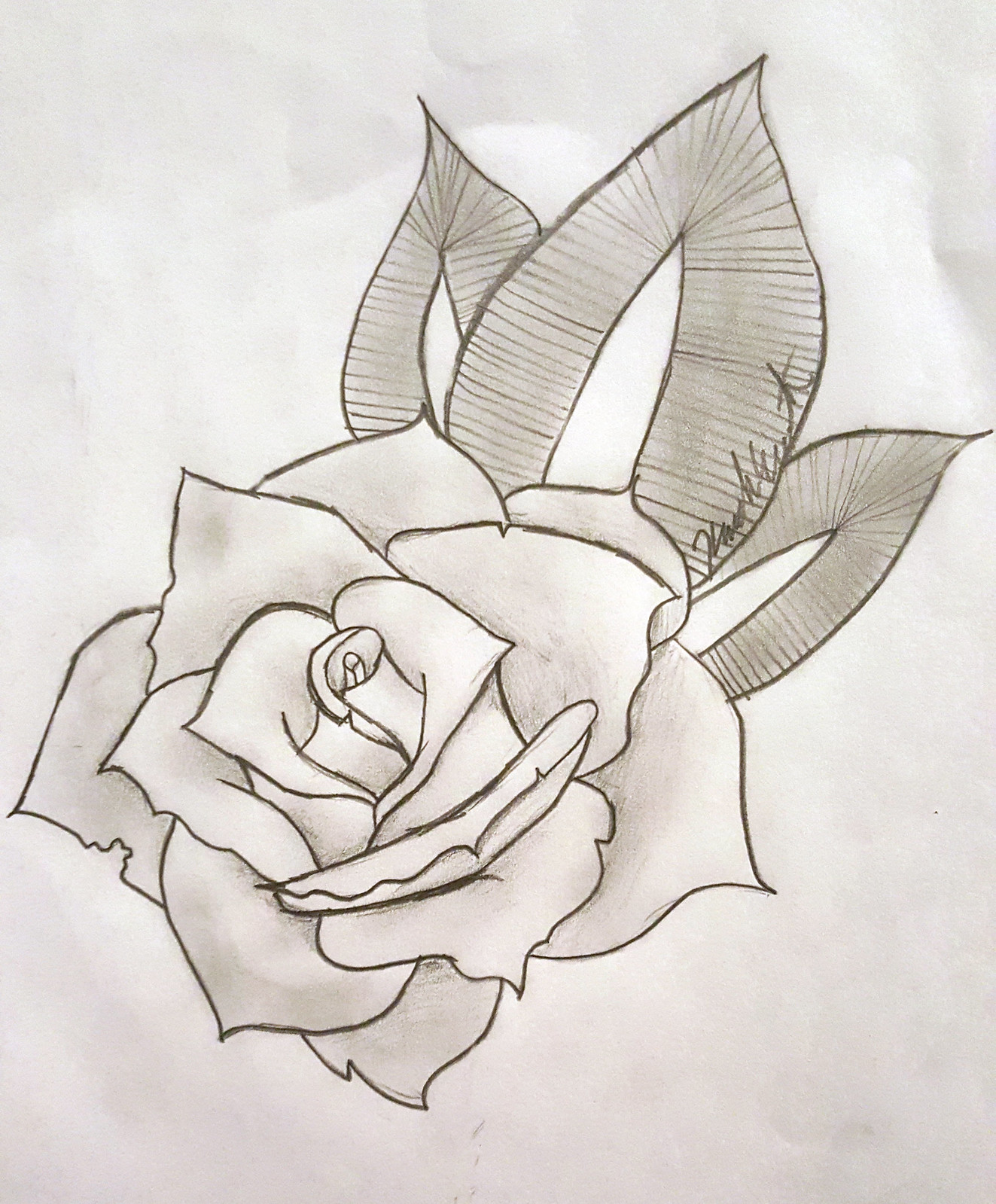This image depicts a detailed pencil sketch of a rose prominently centered on white paper, occupying most of the canvas. The rose, characterized by its tightly closed center and outwardly expanding petals, is drawn with intricate layers that culminate in pointed tips. The petals, which aren't fully open, exhibit subtle pencil shading that provides a gentle contrast to the central bloom. Accompanying the rose are three stylized leaves, marked by dark, heavy pencil outlines and distinct, stripe-like patterns. These leaves display darker shading compared to the rose, with one of them bearing an indistinct signature. The overall sketch presents a realistic portrayal of the rose, while the leaves add an artistic flair to the composition.